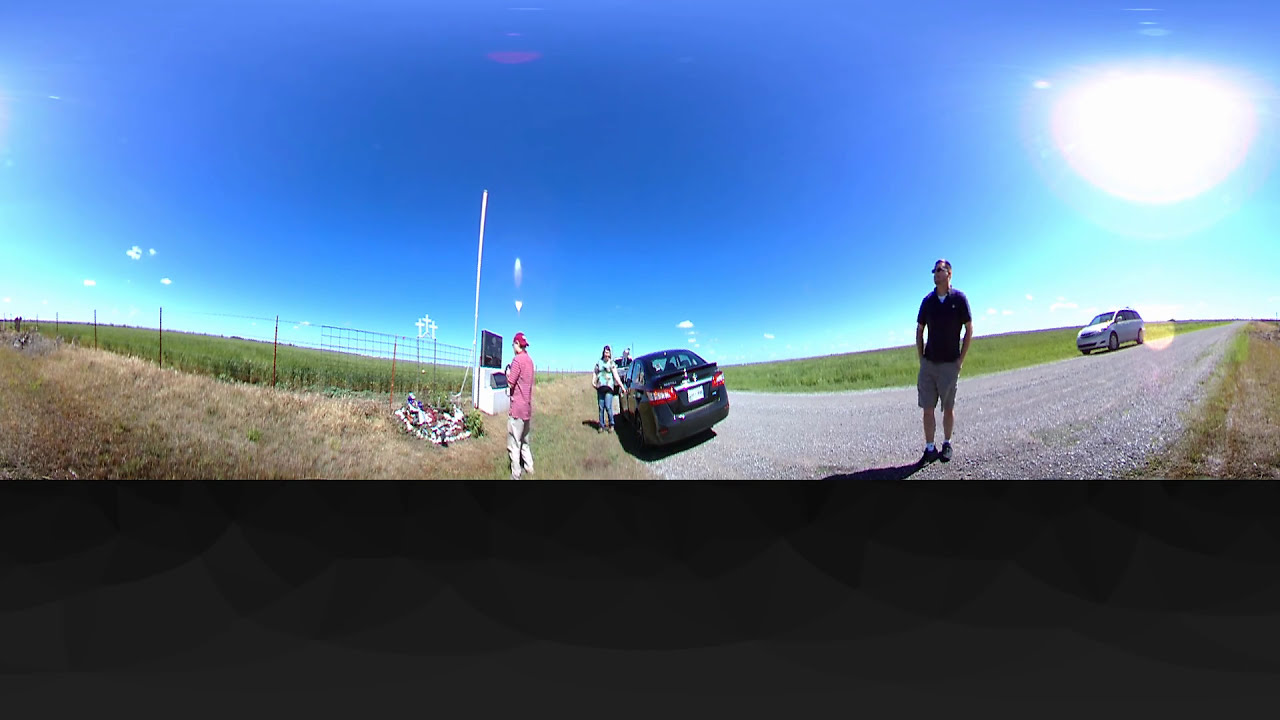The image captures a poignant scene in the countryside beneath a clear blue sky, with the sun shining brightly. It features an unclouded, sunny day with an expansive grassy field, transitioning from vibrant green to patches of tan. The focus is on a roadside memorial signified by three crosses on a fence line, hinting at a tragic event where three individuals may have lost their lives.

To the left, a silver minivan is parked off the gray gravel road. A man in a red and white checkered shirt and beige pants stands by the memorial, looking down at the flowers laid there. Nearby, a woman in a flowered shirt and blue jeans stands near a little black car, opening its passenger side door. Her presence, combined with the arranged flowers, suggest they are paying tribute to the deceased.

Right of center, another man, possibly from the minivan, dons khaki shorts, a dark-colored polo shirt, black trainers with white socks, and sunglasses. He stands solemnly, observing the memorial. Further details include a white pillar with a black sign and a flag post near the flowers, emphasizing the site's significance. All individuals seem engaged in reflective remembrance, highlighting the serene yet somber nature of the scene.